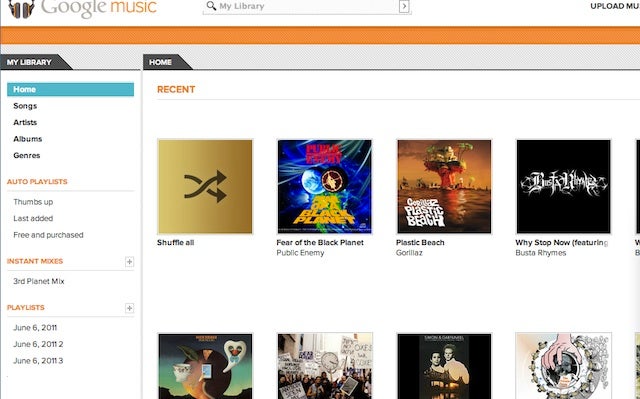This image displays a partially visible web page of the classic Google Music interface, dating back to at least June 6, 2011. In the upper left-hand corner, slightly cut off, the bottom of a pair of traditional over-ear headphones is visible, along with the "Google Music" logo. Dominating the center of the page, a search bar prominently displays the phrase "My Library." To the right of this, the words “Upload Music” are partially visible, truncated by the screen’s cut-off edges, indicating the unfinished capture of the web page.

The left-hand sidebar lists various library categories and options: My Library, Songs, Artists, Albums, Genres, Auto Playlist, Thumbs Up, Last Added, Free and Purchased, Instant Mixes, and specific playlists dated June 6, 2011. Thumbnails representing album art populate the lower part of the left side, with the top-left thumbnail featuring a "Shuffle All" option. The visible ones include recognizable albums such as Public Enemy’s “Fear of a Black Planet” and Gorillaz’s “Plastic Beach,” as well as Busta Rhymes’ single “Why Stop Now.” Other thumbnails present visible artwork, though their titles and artists remain unreadable.

The page is notably incomplete, with portions clipped from the top, bottom, and sides, giving an impression of an archival snapshot rather than a live, functional interface.